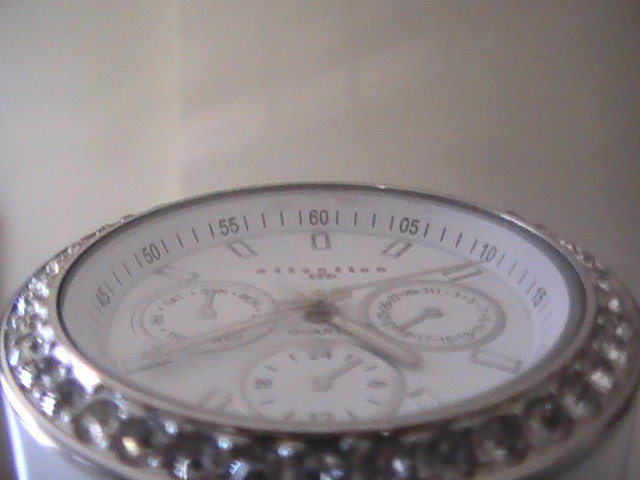This up-close photograph captures the intricate details of a silver wristwatch, albeit somewhat blurry. The watch rests on a white, shiny surface that reflects natural light from the right, casting shadows across the scene. The watch face is white, featuring black numbers and black dashes around the rim to denote the minutes. The brand name, displayed in burgundy font, is slightly blurred but identifiable as reading 'quartz'. The face also includes three smaller circles, each with its own gray hands, indicating additional functionalities such as barometric pressure, moon cycle, and days of the week. The bezel of the watch is adorned with fake diamond-like crystals, adding a touch of elegance. Despite the blur, one can discern the silver watch hands and the time, approximately 4:40 p.m.